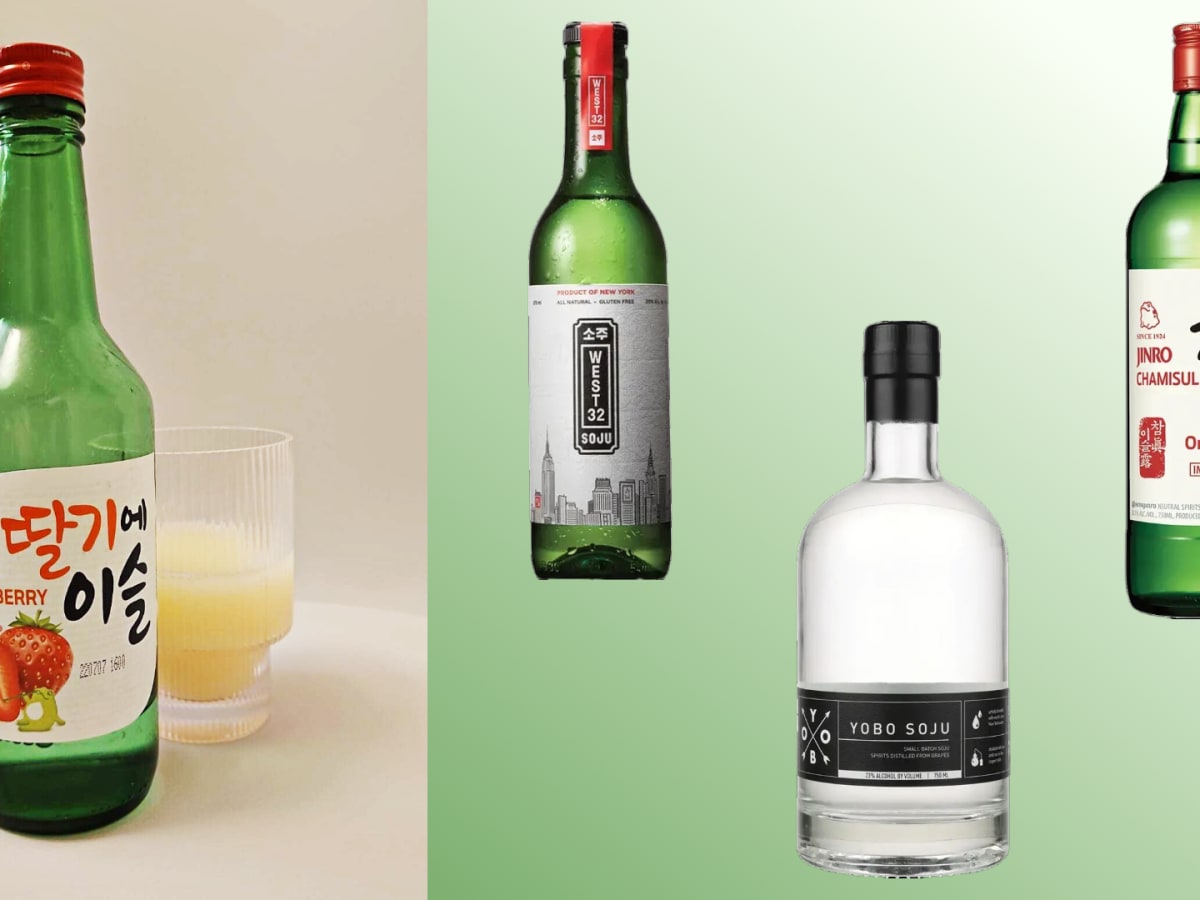The image is a highly detailed advertisement, likely for a Japanese alcohol company, showcasing a collection of four unique beverage bottles with distinctive characteristics against two different background palettes. On the left side of the image, set against a white background, there's a green translucent bottle with a red top and a white label featuring strawberries and Asian script, likely indicating a strawberry-flavored sake or soju. In front of this bottle, a squared-off glass contains an off-white, creamy liquid casting a shadow.

The right side of the image transitions into a gradient from light green pastel to white and features three additional bottles. The bottle on the left, positioned slightly above, is a green translucent bottle with a red, vertically-oriented label and a city graphic on a white and black label—it is labeled "West 32." The central and most prominent bottle is a clear white bottle containing a clear liquid, with a black cap covering part of the neck and a slim black label near the bottom, labeled "Yobu Soju." To the right and at a similar height to the first bottle on this side, there's another green translucent bottle with a red top and a white label with red writing and graphics, labeled "Ginro."

The combined elements of the poster emphasize a premium selection of Japanese-style beverages, potentially flavored sakes or sojus, each with distinct and intricately designed labels, capturing both traditional and modern aesthetics.